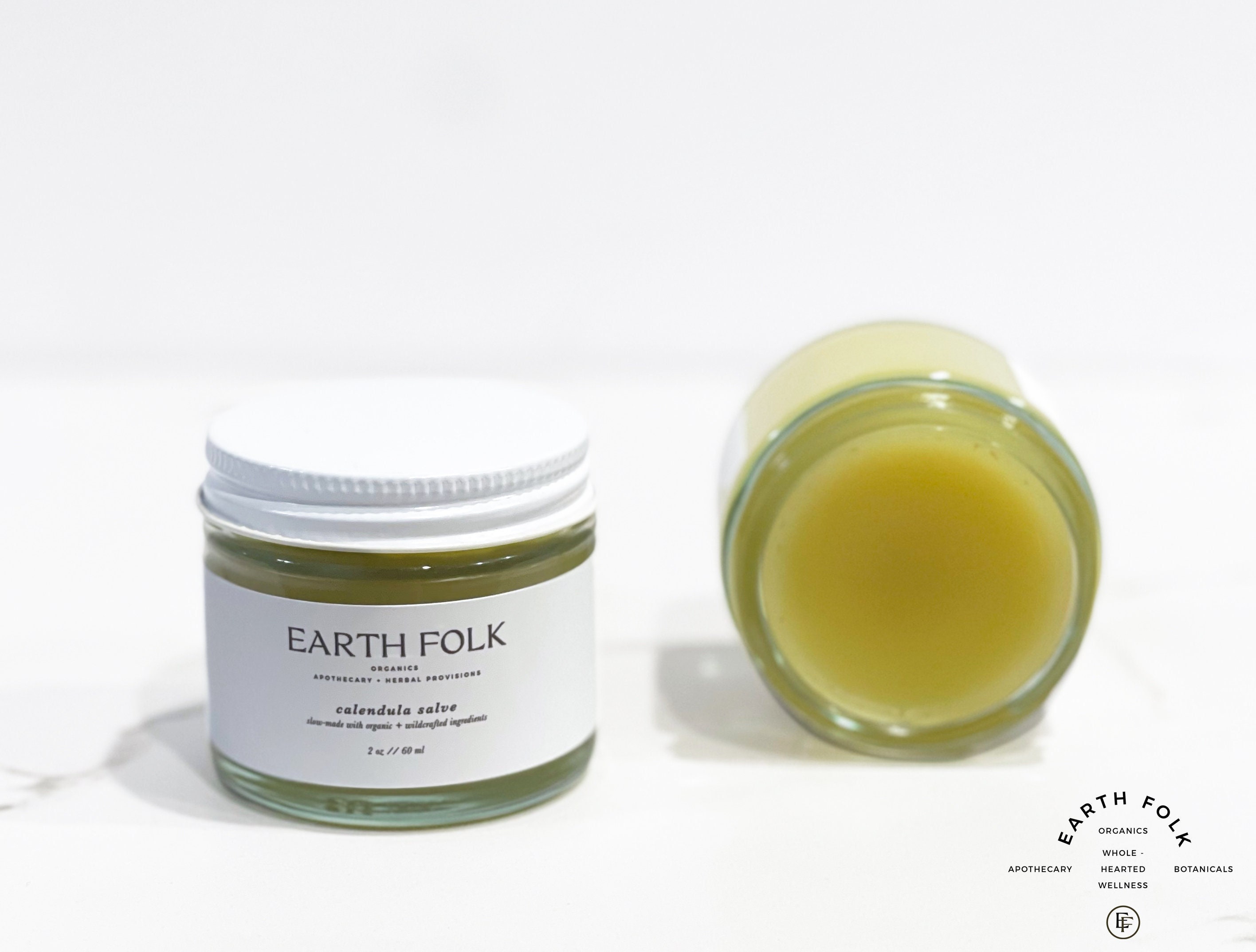The image captures a detailed product shot of a small, squat glass jar with a white screw-on lid, containing a balm-like substance of a yellowish-green, Vaseline-like consistency. The jar prominently features a white label with black text that reads: "Earth Folk Organics, Apothecary and Herbal Provisions - Calendula Salve" along with the quantity, "60 milliliters" (or 2 ounces). Next to the main jar, there's another similar jar laid on its side, showcasing the same greenish-yellow substance inside. The background is white, and at the bottom right corner of the image, a semi-circle watermark displays the text "Earth Folk Organics Wholehearted Wellness," accompanied by a logo with an interlaid 'E' and 'F'. This picture evidently emphasizes the branding and organic nature of the calendula salve product.